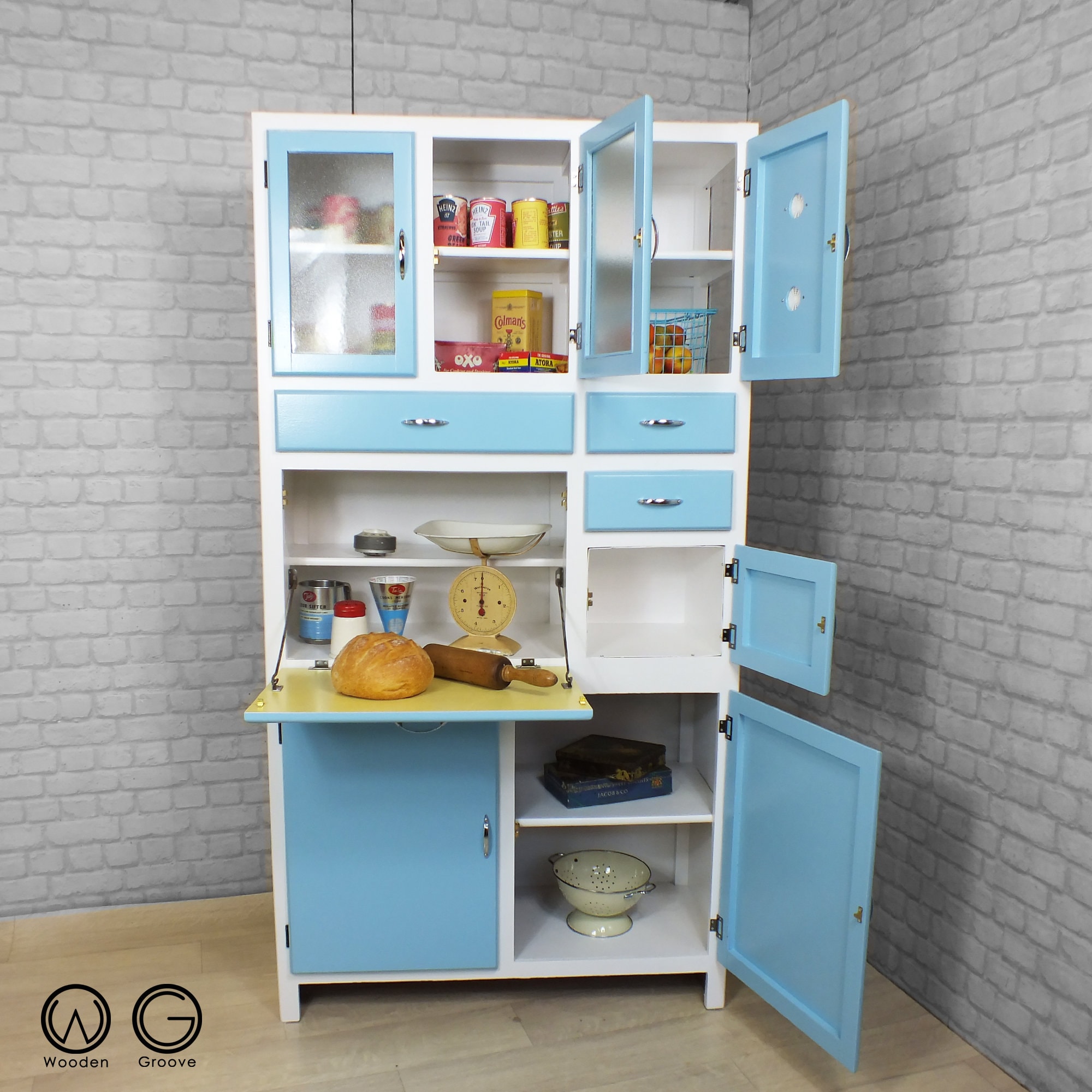This image showcases a beautifully designed, modern pantry cabinet, likely intended as a children's toy kitchen set. The cabinet structure features a combination of fresh white paint and light blue cabinet doors, standing roughly five to six feet tall, four feet wide, and about two feet deep. The pantry is situated against a corner with light wood floors and gray brick-patterned walls. 

The upper section of the cabinet includes glass-fronted rectangular cupboards, some open to reveal various food items like canned goods, soups, and fruits in a basket. The middle section boasts a practical pullout tray painted yellow on the inside, which displays a loaf of bread, a rolling pin, and an old-fashioned food scale. Beneath this are more drawers and cabinets with additional kitchen products such as a colander and various tins and boxes.

A distinctive logo in the lower left corner of the image reads "Wooden Groove," indicating the product's likely brand or design style. The combination of baby blue doors with a white frame, set against a modern backdrop, makes the pantry cabinet both stylish and functional.